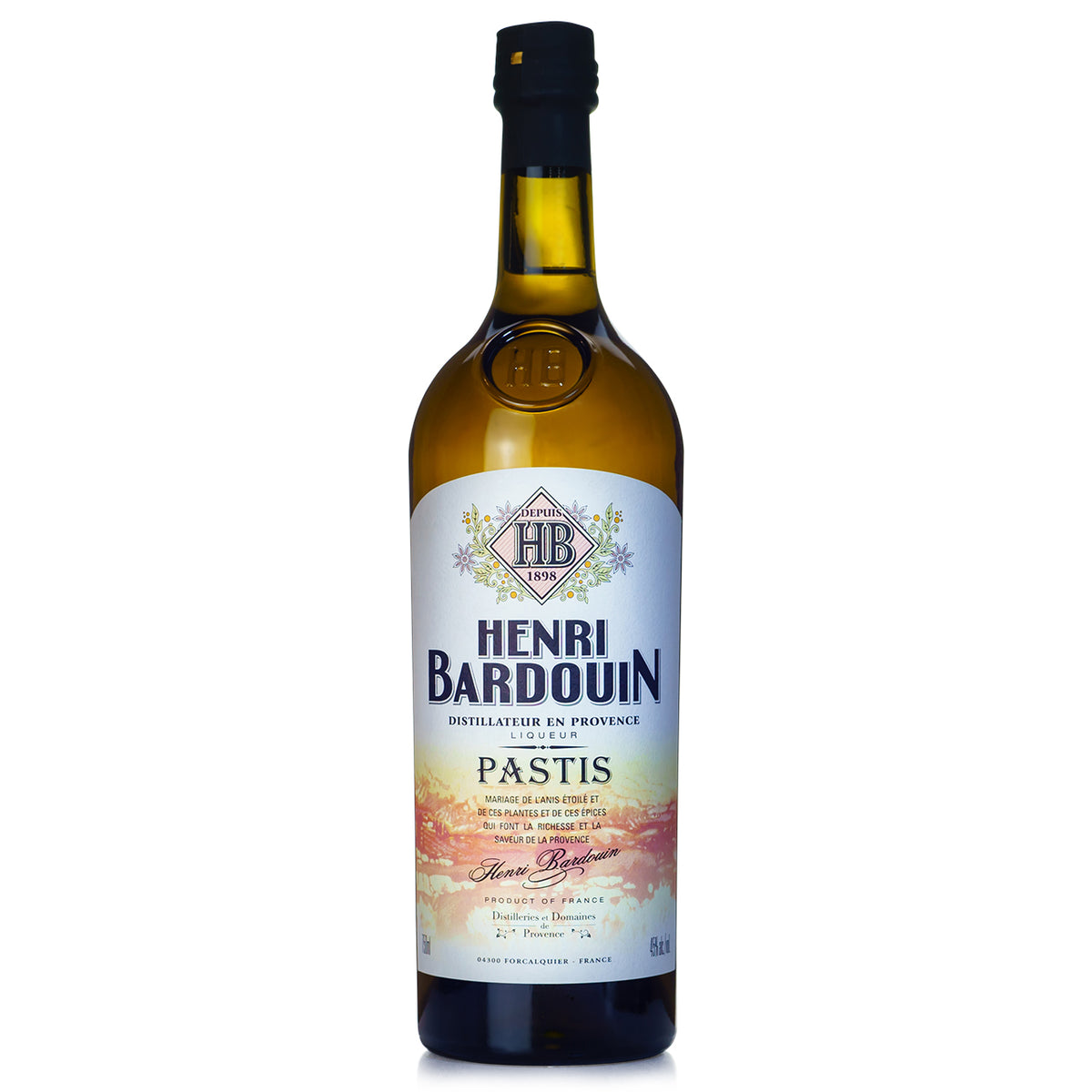The image depicts a solitary bottle against a completely white, colorless background, giving it a sense of blending into a computer screen. The bottle, reminiscent of a wine bottle but distinguished by its darker brown hue, stands tall and narrow with a black cork sealing its top. Prominently featured on the neck of the bottle is an engraved icon "HB" encircled by a ring. The main label on the bottle is predominantly white with colorful designs, including pink lines and floral patterns, enhancing its visual appeal. 

The label includes the following text in different fonts and colors:
- The top of the label features a diamond shape with the inscription "Depuis HP 1898," where the "HP" is highlighted with pink lines.
- Below this, in the largest letters, it reads "Henri Bardouin," the brand name.
- Further down, in smaller letters, it says "Distillateur en Provence Liqueur."
- At the bottom, the word "Pastis" is noted, indicating the type of liqueur.

The overall presentation, including these detailed elements and the combination of floral and colorful touches, makes the bottle visually striking and indicative of a high-quality French liqueur, Henri Bardouin Pastis.